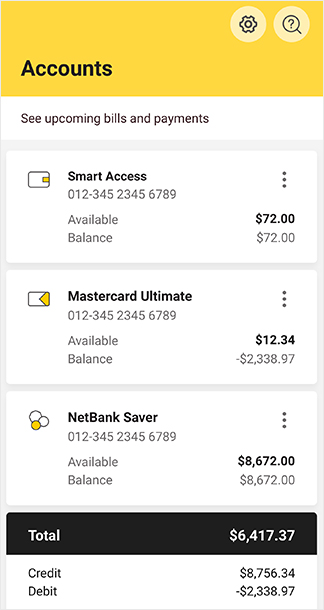The image displays the interface of a mobile banking application in landscape orientation. At the top, a yellow banner stretches across the screen, containing the text "Accounts" along with two icons on the right side: a settings gear and a search magnifying glass. Below the banner, the interface transitions into a white background featuring the header "See upcoming bills and payments."

The screen is segmented into four boxed sections, each detailing different account summaries:

1. **Smart Access:** This box displays a numerical code linked to the account, with labels for "Available" and "Balance," both showing amounts of $72.00.
2. **MasterCard Ultimate:** Similar to the first, this box includes a numerical code, with "Available" listed as $12.34. The "Balance" indicates a negative amount of -$2,338.97. 
3. **NetBank Saver:** This box also contains a numerical code, with both "Available" and "Balance" showing $8,672.00.
4. **Total Overview:** The final box, distinguished by a black header, shows a "Total" of $6,417.37. Below this, it details "Credit" as $8,756.34 and "Debit" as -$2,338.97.

Each section efficiently presents the financial statuses of the various accounts linked to the user’s mobile banking app.